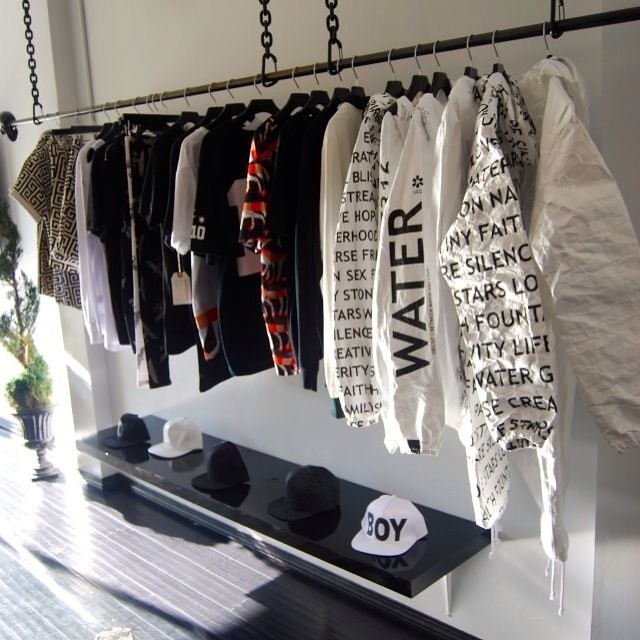In this detailed photograph of a stylish indoor setting, likely either a small boutique or an organized closet, a central silver rod is prominently featured. The rod, suspended by black chains, secures several silver hangers. Neatly arranged jackets and shirts are displayed on these hangers, showcasing a gradient of colors: lighter shades on the right, medium red hues in the center, followed by darker shades toward the left. Below the hanging garments, a glossy black shelf holds a row of five caps organized from left to right: a black cap, a white cap, two additional black caps, and another white cap emblazoned with the word "BOY" in large letters. Adding a touch of nature, a large indoor plant in an urn is visible in the background on the left, complementing the organized and trendy atmosphere of the scene.